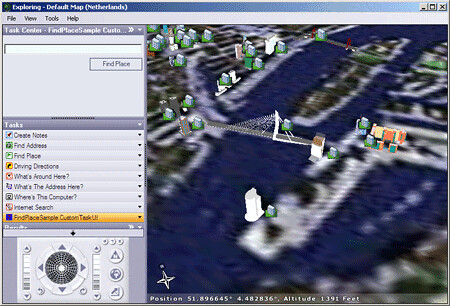This is a detailed screenshot from a map program. On the right side, the map is dominated by a large body of water, depicted in deep blue hues that clearly differentiate it as such. In the center of the image, a bridge spans across the water, connecting two segments of the city. Scattered around the map are several white models of buildings, notable for their brown roofs. Additionally, a distinct bright orange building stands out on the right side of the map. On the left side, the map displays various green models which could represent either buildings or trees. Furthermore, the left side of the screen contains a legend, though it's difficult to read due to the small size of the image. Finally, in the bottom left corner, there's a control panel that users can presumably use to navigate the map.